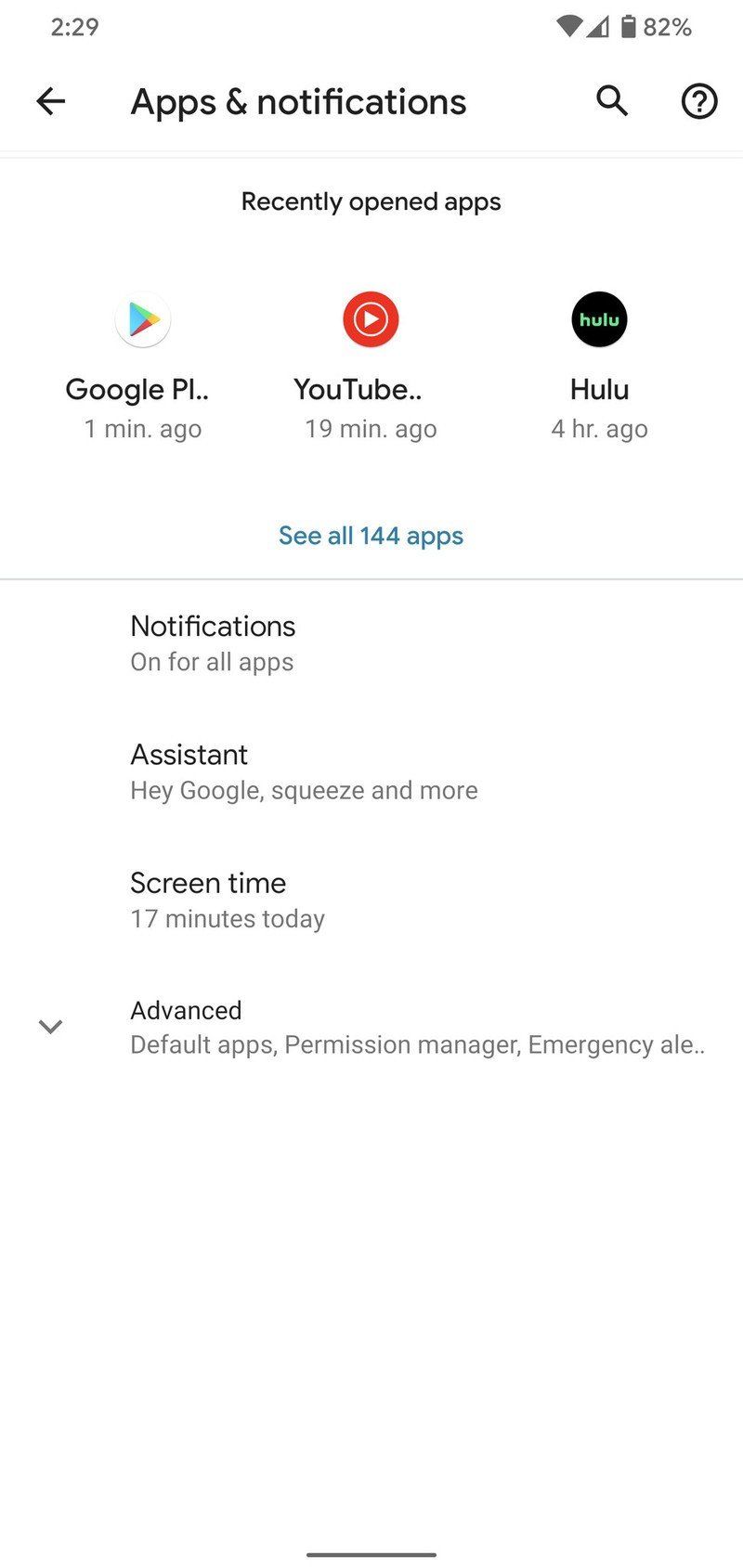This image captures a screenshot of a smartphone's "Apps & Notifications" settings. At the top left corner, a notification icon indicates there are 229 notifications, while the top right corner shows the battery level at 82%. Beneath the notification bar, "Apps & Notifications" is typed in black within the search bar. Below that, the section labeled "Recently Opened Apps" displays three apps horizontally.

The first app, "Google," was accessed one minute ago, accompanied by its icon—an uppercase 'G' in Google's signature colors. Next, the "YouTube" app was opened 19 minutes ago, identifiable by its red circle icon with a white play button and a smaller white circle within the red circle. The third app, "Hulu," was last used four hours ago, represented by its green logo spelling "Hulu."

Following this listing, a blue text prompt invites users to "See all 144 apps." Underneath, a summary section indicates that notifications are enabled for all apps, with a mention of "Assistant, Hey Google, Squeeze," among other functionalities. Additionally, the screen time is logged at 17 minutes per day. At the bottom, an "Advanced" category includes options for "Default Apps," "Permission Manager," and "Emergency."